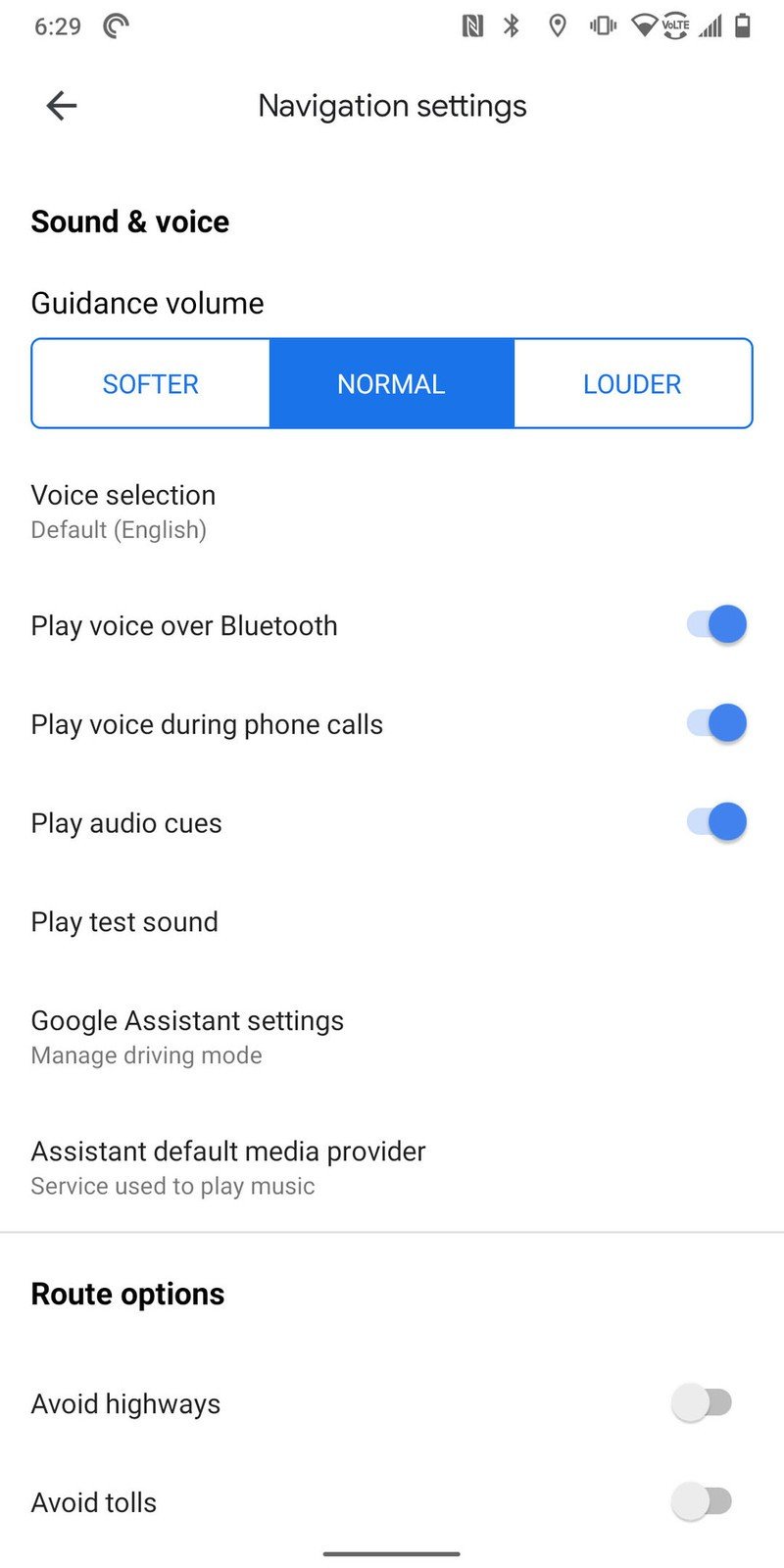Here is a cleaned-up and detailed caption for the image based on the provided voice description:

---

**Screenshot of Navigation Settings on a Smartphone (Timestamp: 6:29 PM)**

The image showcases the detailed navigation settings on a smartphone. Key settings displayed include:

1. **Closed Captioning**: Enabled.
2. **Bluetooth**: On and connected to other devices.
3. **Google Location Services**: Activated (indicated by the icon on the upper right-hand side).
4. **Vibration Settings**: Enabled.
5. **Battery Status**: Approximately 50% charged.
6. **Signal Strength**: Full bars.
7. **VoLTE Settings**: Active.
8. **Wi-Fi**: Connected with a medium to strong signal.

**Navigation Audio Settings**:
- **Guidance Volume**: Set to 'Normal' (other options include 'Softer' and 'Louder').
- **Voice Selection**: Default English.
- **Play Voice Over Bluetooth**: Enabled.
- **Play Voice During Phone Calls**: Enabled.
- **Play Audio Cues**: Enabled.
- **Play a Test Sound Option**: Available.

**Google Assistant Settings**:
- **Manage Driving Mode**: Available.
- **Assistant Default Media Provider**: Set to a service used to play music.

**Route Options**:
- **Avoid Highways**: Disabled.
- **Avoid Tolls**: Disabled.

This comprehensive settings menu illustrates the various configurable options available for navigation, audio cues, and connectivity preferences on a smartphone, highlighting the customization available to tailor the user's navigation experience.

---